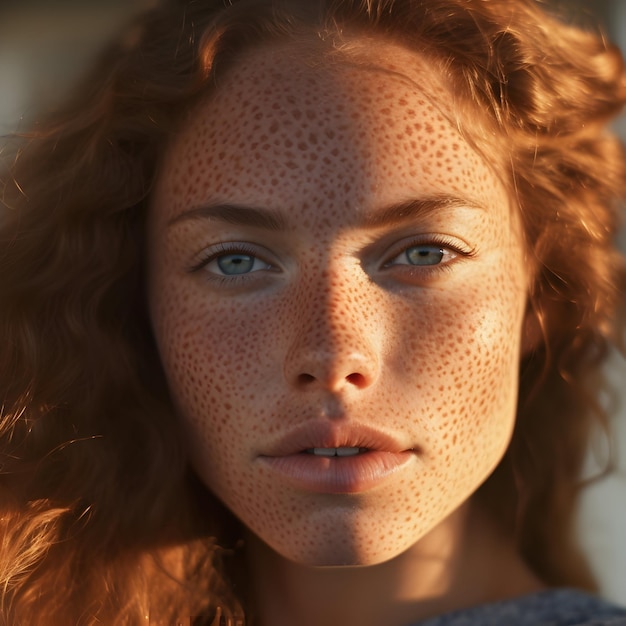The image depicts a young woman with flowing red curly-wavy hair caught in the wind, illuminated by sunlight from the right side. She has striking light blue eyes, full light pink lips slightly parted to reveal her top two teeth, and reddish-brown eyebrows with medium-length eyelashes. Her light-colored skin is covered with what appears to be an unusual pattern of freckles or large brown spots, adding an uncanny, almost AI-generated quality to her otherwise realistic appearance. She wears a gray sweater and looks very serious, perhaps similar to a model. The sharp focus on her face contrasts with a slightly blurred neck and hair, enhancing the ethereal effect.